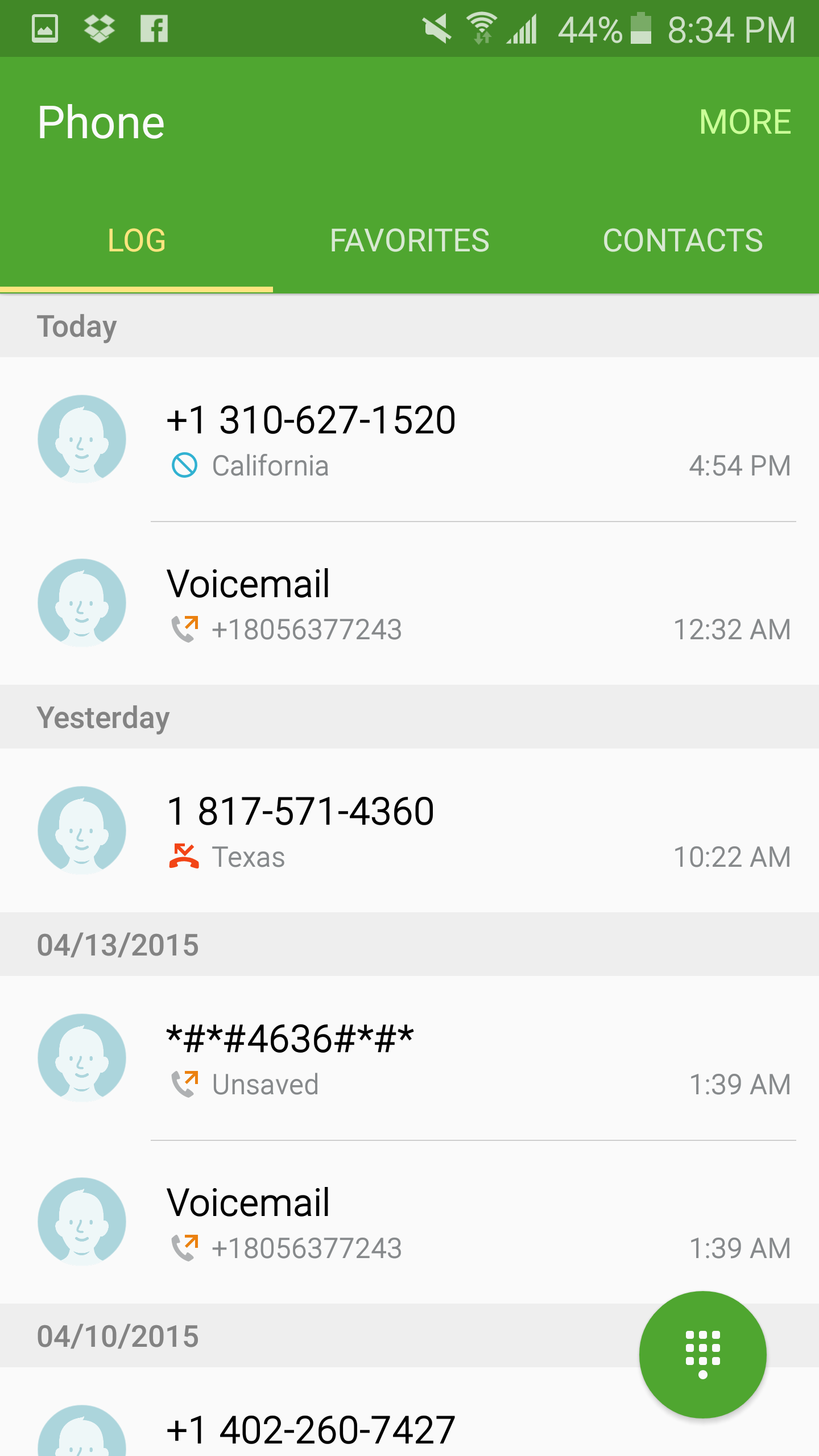This is an image of a smartphone screen displaying a phone app interface. At the top center of the screen, there is a green rectangular box with various phone app icons. Below this box, there are three main tabs labeled "Log," "Favorites," and "Contacts," with an additional "More" option on the far right.

The "Log" tab is currently selected, indicated by a yellow underline beneath it. The log displays recent call activity, with sections organized by date. Today's log includes two entries: one from a blocked number in California and another from voicemail. The log for yesterday shows a missed call from Texas. Further down, there are entries from April 13, 2015, including another voicemail and an unidentified number.

At the top of the screen, different icons are visible, including a photo, a Jeep icon, a Dropbox icon, and the Facebook icon, lined up from left to right. On the far right side of the screen, system icons display the phone's current status: a mute or volume-off icon, the network signal icon, the Wi-Fi connectivity icon, the battery level at 45%, and the current time, which is 8:34 PM.